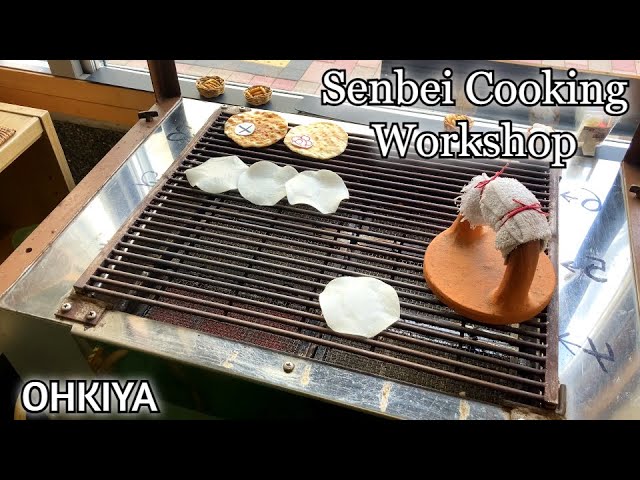This detailed photograph captures the Okiya Senbei Cooking Workshop, offering a top-down view of a rustic grill set on a steel table framed by wood. Bold white text with black outlines reads "Senbei Cooking Workshop" at the top left, while the bottom left corner displays the word "O-H-K-I-Y-A." The grill top, which features numbers 1 to 6 along its sides, showcases several white, flat, circular senbei, resembling small tortillas. These senbei are placed both flat and folded on the grill surface. At the bottom right of the grill, there's a wooden-handled press with a cloth tied around it. Additionally, two crispy, brown senbei rest at the back of the grill. The top of the frame includes a windowsill with two danishes or treats and a small outward-facing sign in the top right corner, all adding to the detailed culinary scene.